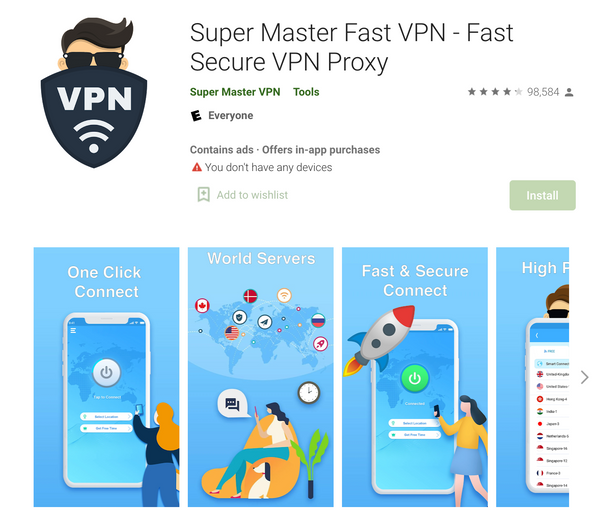The image appears to be a screenshot taken most likely from a tablet device, given its horizontal orientation. It showcases an application interface for "Super Master Fast VPN," a VPN service. The app is titled "Super Master Fast VPN: Fast & Secure VPN Proxy" and is developed by Super Master VPN. It currently has a rating of 4 out of 5 stars based on 98,584 user reviews. The application is free to download but includes advertisements and offers in-app purchases. At the bottom of the screen, there are various icons depicting the app's features such as "One-Click Connect," "World Servers," "Fast and Secure Connect," and an additional feature that is partially visible, likely labeled "High-Speed" or similar.

The app is not installed on the user's device, and they have the option to add it to their wishlist. The logo features a character with brunette hair and sunglasses, peeking over a shield that displays the text "VPN" along with a Wi-Fi symbol, enhancing the visual appeal and branding of the application.